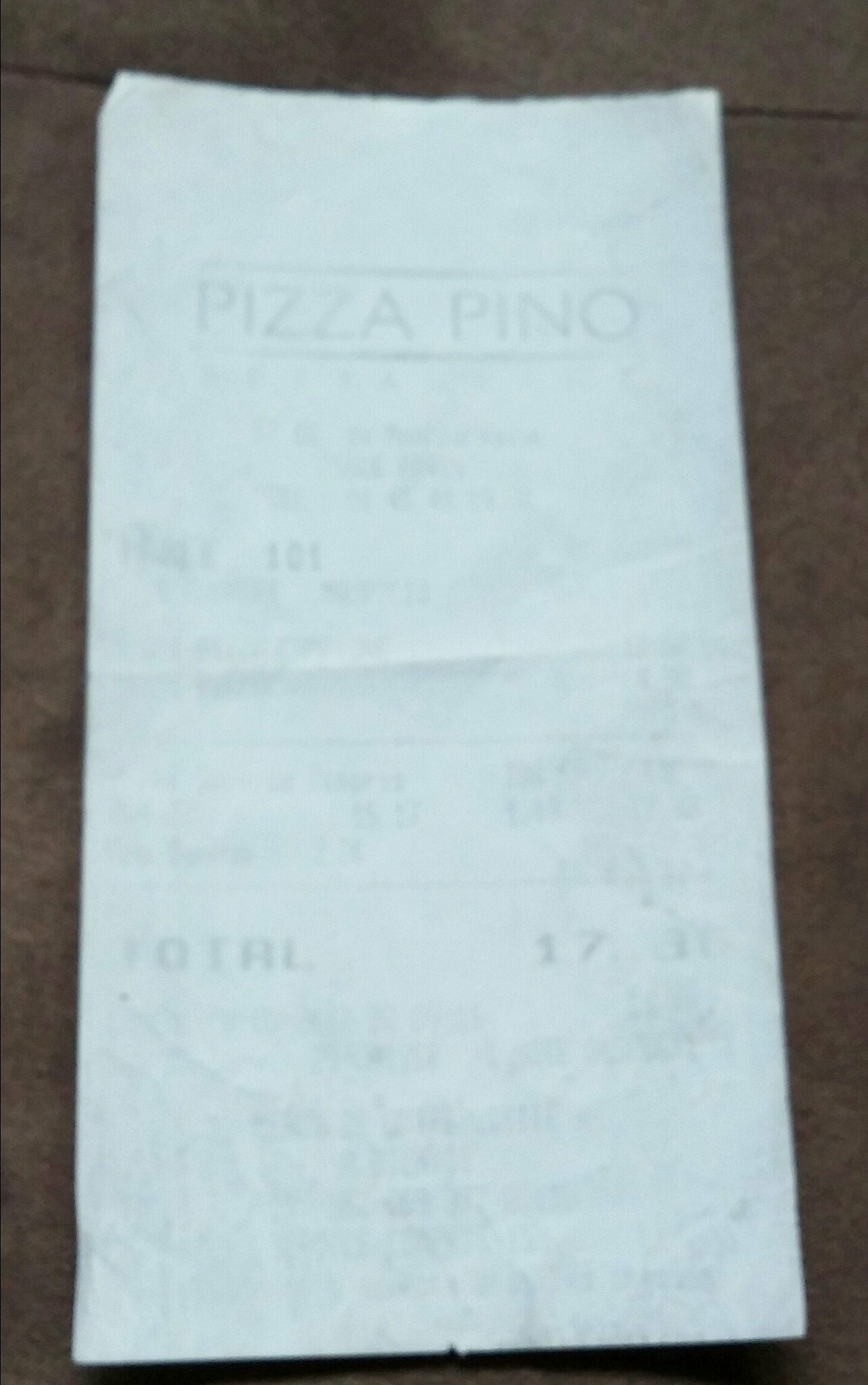The image displays a very old and faded white receipt from a place named Pizza Pino, evident from the all-caps black text, "PIZZA PINO," at the top, underlined and overlined by black lines. The receipt, crumpled and worn, shows significant signs of aging, making most of the text almost illegible, except for a few key details. The total amount at the bottom appears to be $17.30, though the change is hard to discern due to the blurriness and low resolution of the photo. The receipt rests on a dark, textured surface, possibly a concrete floor or a granite-like countertop. The rectangular receipt is oriented vertically in the image, further emphasizing its faded condition and the difficulty in reading its details.